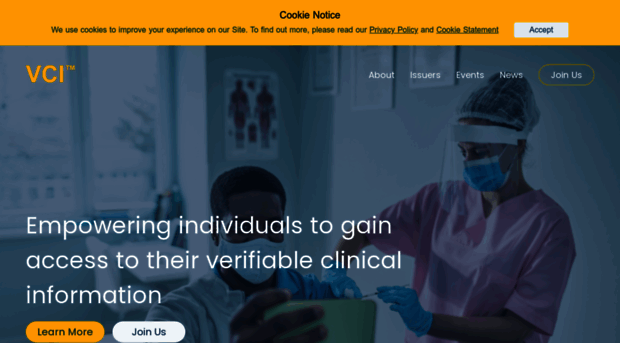The image displays a website interface. At the top, a goldenrod yellow banner features prominently, with the text "Cookie Notice" in bold black font, both "C" and "N" capitalized. Below this heading, the banner states, "We use cookies to improve your experience on our site," with "site" also capitalized. Further information is available by clicking on the underlined phrases "privacy policy" and "cookie statement." An "Accept" button is present beneath this message.

The main part of the website appears to showcase a graphic of a medical office or clinical environment. In the top left corner, the same goldenrod yellow color is used to display the acronym "VCI." To the right, the navigation menu includes options: "About," "Insurers," "Events," "News," and "Join Us." Further down, a tagline reads, "Empowering individuals to gain access to their verifiable clinical information." Two buttons are present below this text: one yellow button labeled "Learn More" and another white button with black text labeled "Join Us."